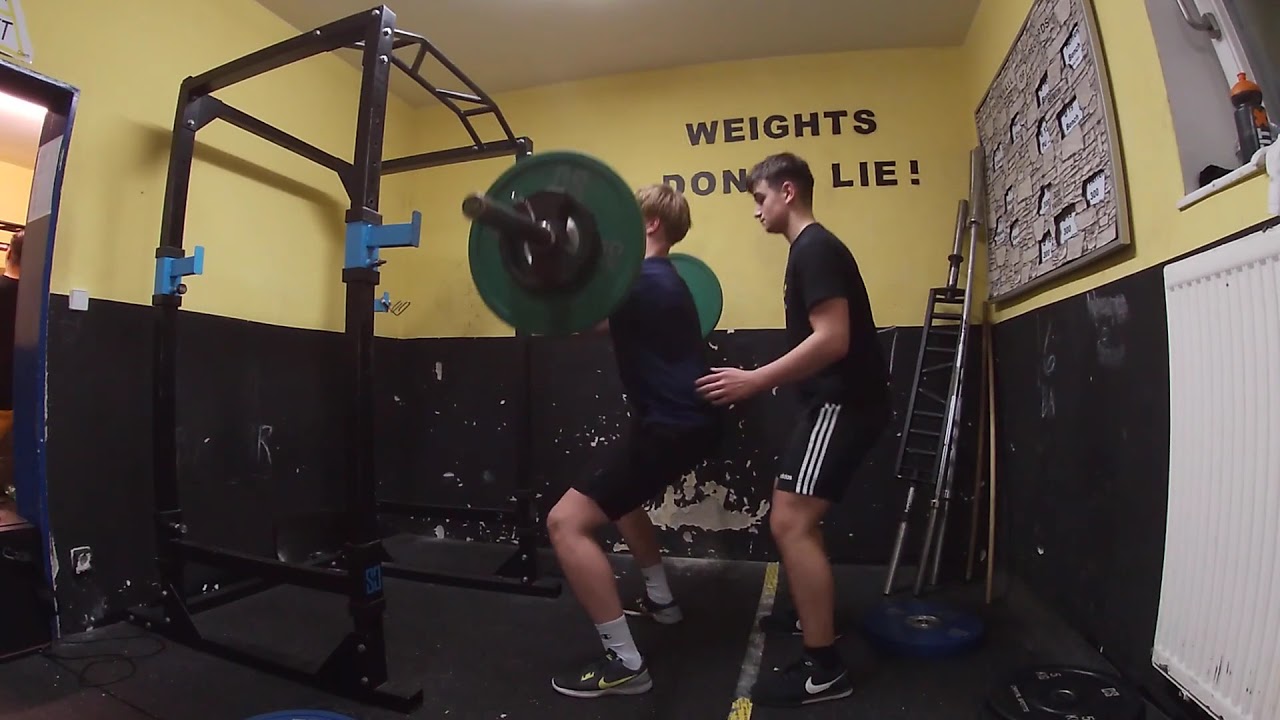The image captures a scene in a small high school gym, characterized by its prominently yellow and black walls, with notable areas of erosion revealing tan drywall underneath. Central to the image are the words "weights don't lie!" boldly painted in black on the yellow section of the wall. In the middle of the frame, two young males are engaged in a weightlifting exercise. The lifter, dressed in black shorts, white Nike socks, Nike shoes, and a short-sleeved black shirt, is attempting to lift a barbell with two green weight plates. His spotter, wearing shorts with three white stripes, black socks, Nike shoes, and a black short-sleeved shirt, stands close behind, prepared to assist. The gym's floor is covered with a rubber mat, and behind the pair, there is a wall-mounted bulletin board cluttered with notes, a framed picture, and a plaque. Additionally, a windowsill with a sports drink sitting atop it is partially visible, along with a section of white wall.